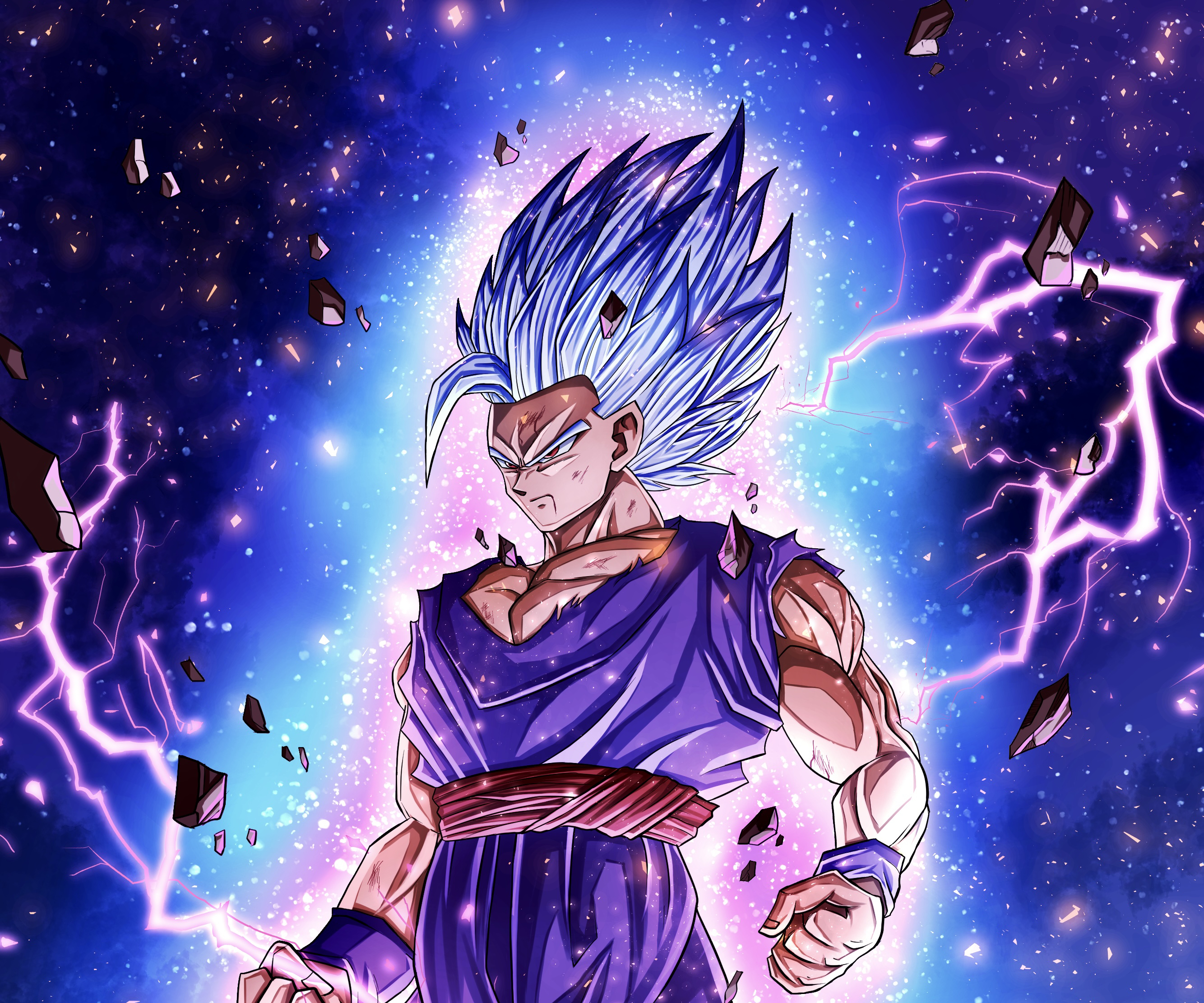The image depicts Gohan from Dragon Ball Z in an intensely dramatic scene. Gohan, a highly muscular and medium-skinned male anime character, stands centered in the frame, exuding an aura of formidable energy. His long, spiky, blue hair with black tips is electrified, standing straight up and flowing upwards, with one rebellious lock pointing towards his face at nose level. His countenance is one of fierce determination and palpable anger, with clenched fists ready for battle.

He is clad in a torn, sleeveless purple tunic with a brown belt cinched just below his chest. His attire has clearly seen better days, evident from the ripped sleeves and the scratches all over his muscular arms, chest, and forehead. Blood trickles from the side of his mouth, further emphasizing his relentless fighting spirit.

The backdrop is a surreal outer space scene, filled with a starry expanse and floating asteroids, enhancing the ethereal and otherworldly atmosphere. Gohan is enveloped in a brilliant aura of purplish-pink light, transitioning seamlessly into a captivating blue glow. Lightning crackles menacingly around him, with bolts seemingly emanating from his form and shooting skywards, adding to the visual spectacle.

In this electrifying scene, Gohan embodies the epitome of power and resolve, set against an explosive cosmic battlefield.